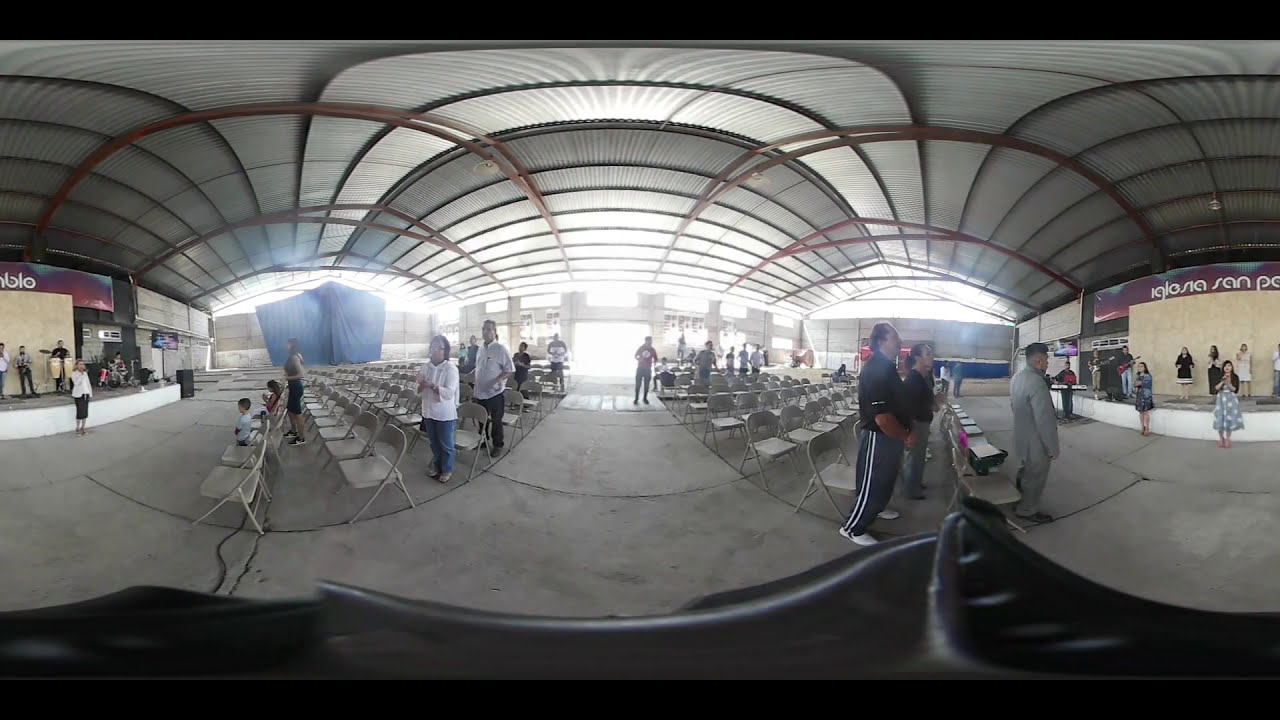This indoor photograph captures a panoramic view of a community gathering, potentially at a civic center or a place where community meetings are held. It appears to be a composite image, stitched together to create a rounded, 360-degree effect, resulting in a slightly warped and spherical perspective. The image shows two sets of rows of light gray, foldable metal chairs arranged in symmetry—one set on the left and one on the right. In the foreground on the right, there is a man dressed in sweatpants or workout pants featuring two white stripes, accented with tan, gray, and blue colors.

To the right side of the image, a raised stage is visible. In front of this stage, two women are singing, accompanied by a man playing an electric piano or keyboard. On the stage, two men are playing guitars, joined by three or four additional singers. On the left side of the image, the other half of the stage is visible, featuring a woman in a white sports jacket and black skirt singing into a microphone. Behind her, a band is seen with a person playing bongo drums, another on a traditional drum set, and additional musicians whose instruments are partially obscured.

In total, there are about 25 to 30 people scattered throughout the room, with several standing, possibly engaged in some formal activity like the Pledge of Allegiance. The room's floor is a light gray concrete, and the ceiling is architecturally unique with overlapping arch-shaped wooden supports. Natural light filters in through windows and doors in the background, adding a soft, inviting glow to the scene. On the far right wall, partially visible letters spell out "B-L-O," and there is a hint of additional writing above that may read "Iglesias San Pablo." The image is bordered by a black header and footer, enhancing the bubble effect.